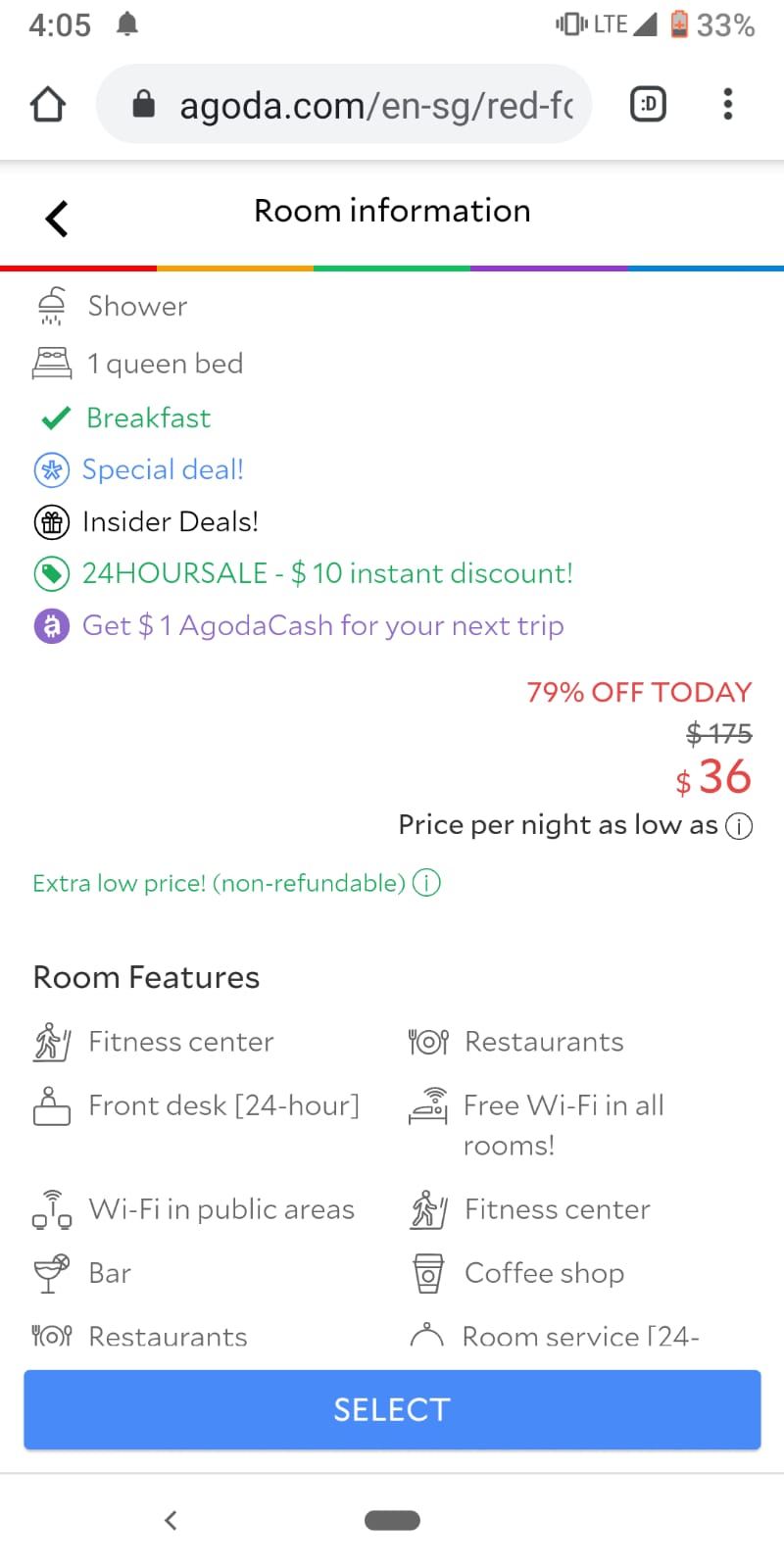**Caption:**

This detailed screenshot from a smartphone, likely captured from a website, features a white background interface. At the very top, indicators show the time as 4:05, a bell icon, battery percentage at 33%, and LTE connectivity. Below this is the website URL "agoda.com/en-sg/red-f..." accompanied by navigational elements including a back arrow, a horizontal ellipse with a padlock icon, a black square, and three vertical dots.

A light gray separator line follows, leading to the main section labeled "Room Information" in black text, centered and flanked by a back arrow on its left. Underneath, a multicolored line transitions through red, yellow, green, purple, and blue. Relevant room details follow, including a shower icon with the word "shower" beside it, a bed icon with "one queen bed" to its right, and a green check-marked "breakfast."

Available offers and deals are prominently listed:
- A "Special Deal" in light blue with a blue star icon.
- "Insider Deals!" with a symbol resembling a gift box.
- "24-hour Sale - $10 Instant Discount!" in green, marked with a green circle.
- In purple, the offer "Get $1 Agoda Cash for Your Next Trip."

Pricing details include a striking red "79% off today," showcasing a crossed-out price of $175 now reduced to $36, with a note about the price being per night.

Located on the left side is a green label, "Extra Low Price, Non-refundable," with a green eye icon. Below room features are organized into two columns, each with corresponding icons:
- Left column: Fitness Center (treadmill), 24-hour Front Desk (person behind a desk), Wi-Fi in Public Areas (Wi-Fi bars), Bar (cocktail glass), Restaurants (restaurant table).
- Right column: Restaurants (plate with fork and spoon), Free Wi-Fi in All Rooms (Wi-Fi bars), Fitness Center (treadmill), Coffee Shop (coffee cup), Room Service 24-hour (bell icon).

Finalizing the details, a prominent blue button at the bottom reads "Select" in white letters.